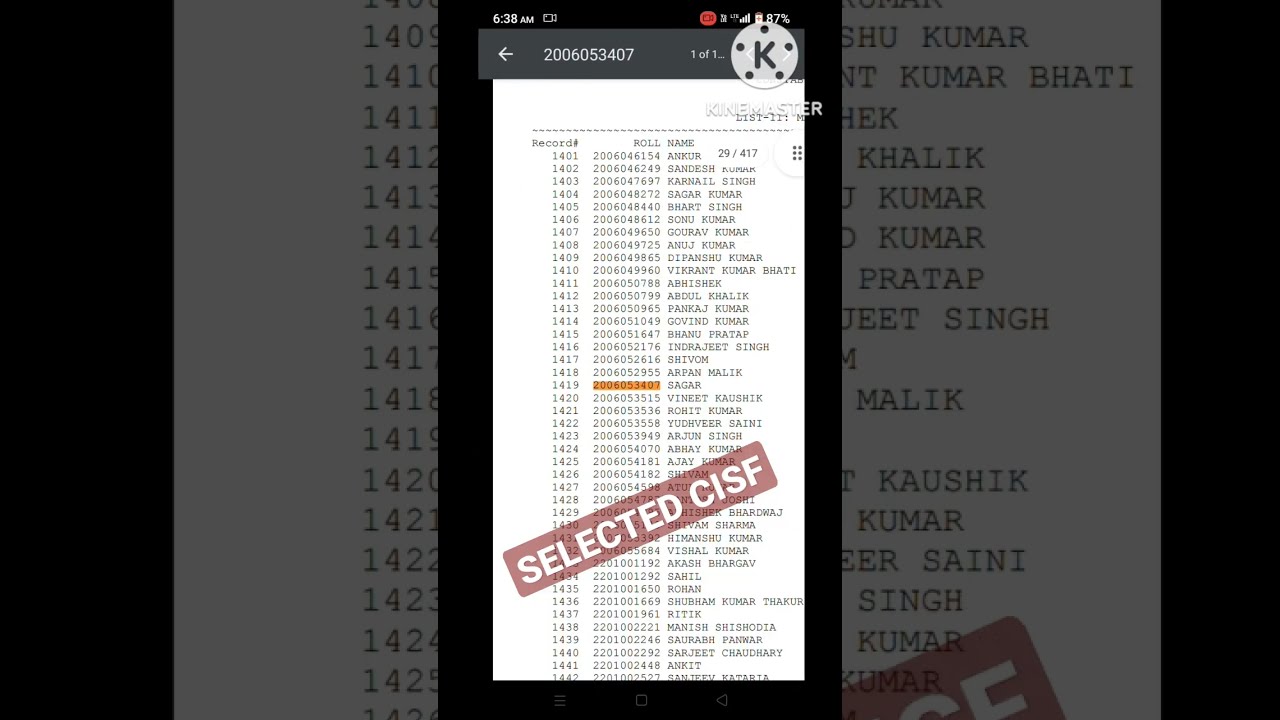The image is divided into three vertical sections, with the first and third sections showcasing darkened close-ups of the middle section. The middle section contains a screenshot of a phone app displaying a PDF file. At the top, we see the notification bar showing the time as 6:38 AM, signal strength, and the battery at 87%. On the top right corner, there's a watermark from KineMaster, featuring a circled "K". The PDF title, "2006-053-407," is situated in a dark gray bar, with navigational arrows and "1 of 1" text beside it. The document lists numbers and names in columns labeled 'Record Number', 'Roll', and 'Name', with the text in black on a white background. Among the South Asian or Indian names and numerical entries, one roll number is highlighted in the center. Over this part of the image is a red banner that reads "SELECTED CISF".